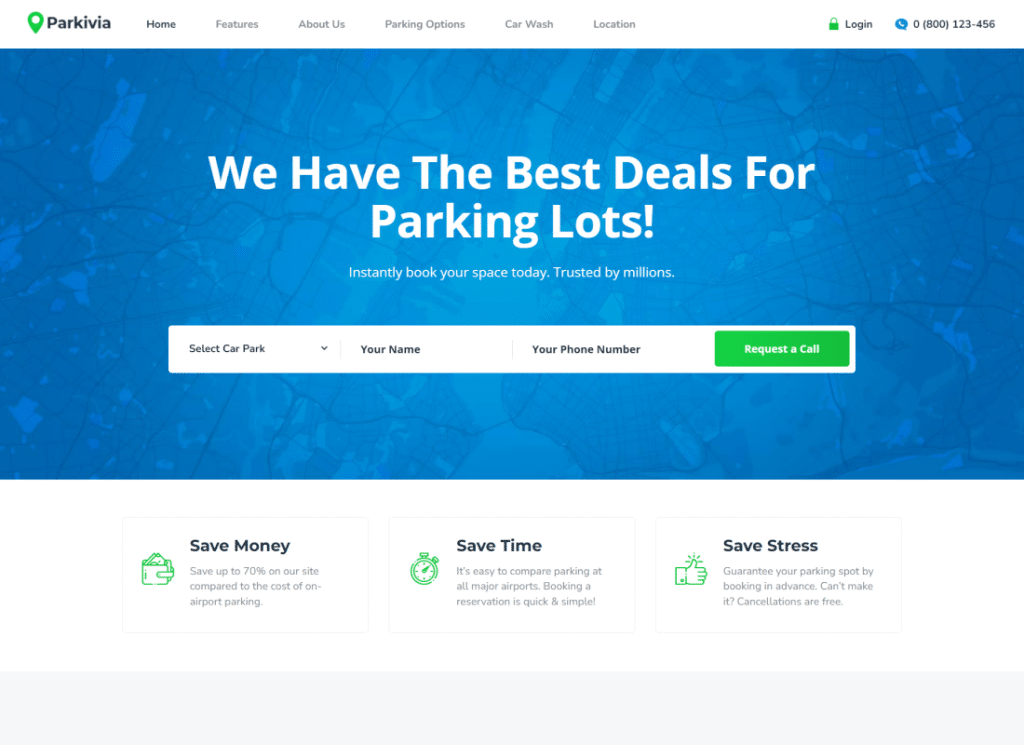The image is a left-to-right horizontal screenshot from a web page featuring a clean, minimalistic design with prominent white space derived from the computer screen background. At the top left corner is a small green icon followed by the bolded black text "Parkivia." Adjacent to this is a navigation menu listing "Home" (in bold), "Features," "About Us," "Parking Options," "Car Wash," and "Location." 

On the upper right corner, there is a padlock icon next to the text "Log In," a phone icon, and a phone number for customer support. Below the navigation bar is a visually appealing shaded blue background with diagonal lines. Centered on this background in large, bold white text are the words, "The Best Deals for Parking Lots." 

Underneath is a smaller font text that reads, "Instantly Book Your Space Today, Trusted by Millions." Beneath this are white text fields labeled "Select Car Park," "Your Name," and "Your Phone Number" in black font, all housed within a long, thin rectangular box. Adjacent to this form is a green button with white text that says, "Request a Call."

Further down, three lightly gray-outlined boxes each contain an icon and black headings which read: "Save Money," "Save Time," and "Save Stress." Beneath each heading is a brief description expounding on how the service helps users save money, time, and reduce stress.